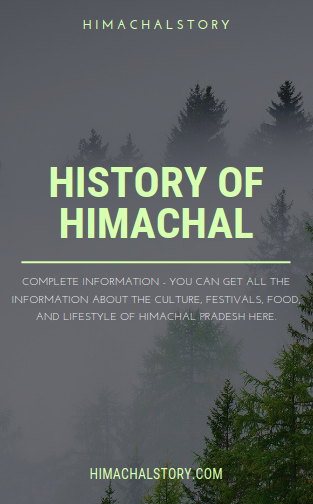The image is a cover page that prominently features a foggy, misty forest backdrop, with gray skies. The treetops, possibly pine or evergreen, are barely visible through the dense fog, mainly concentrated on the top and right side. In contrast, the lower right corner displays clearer, more visible green trees. 

At the top of the image, in chartreuse-colored text, it reads "H-I-M-A-C-H-A-L-S-T-O-R-Y," followed by "History of Himachal" in the center, with the same color. Below this, a horizontal green line separates a white text block that reads, "Complete information. You can get all the information about the culture, festivals, food, and lifestyle of Himachal Pradesh here." Finally, at the bottom, in chartreuse text, it displays the website "HimachalStory.com."